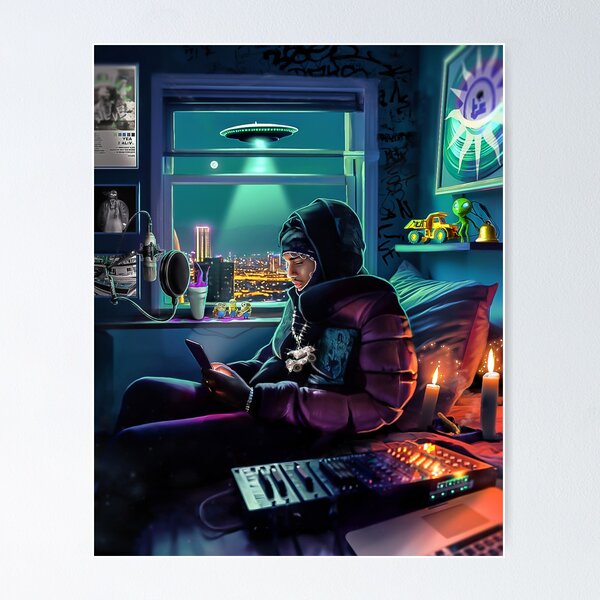The image is a highly detailed, likely AI-generated, science fiction scene. It depicts a man dressed warmly in a purple down jacket with a hood over a hooded garment, gloves, a scarf, a hat, and a ski mask, sitting on a bed or chair in a dimly lit room. He's engrossed in his phone, his face illuminated by the screen, suggesting perhaps he's texting. Around him, two candles flicker, casting a warm yellow glow, hinting at a power outage.

The room is cluttered with various items: an ashtray with a smoking item, an electronic DJ mixing board next to a computer, and multiple other gadgets. A recording microphone is also visible within the scene. Decor on the walls includes multiple posters and writings, with one particularly vague sun-like image. On the window sill, there are small figurines, potentially minions, an alien toy, and a truck. 

Through an adjacent window, an otherworldly, nighttime cityscape is visible, dominated by the moon and an alien spaceship casting a beam of light down over the city, the light reflecting subtly into the room. The overall ambiance is dark and mysterious, filled with a mixture of technology and sci-fi elements.